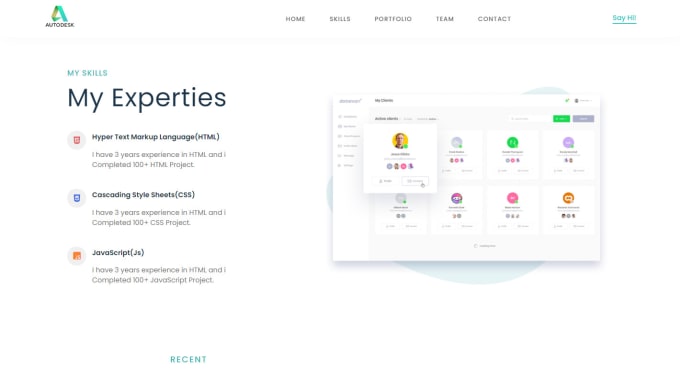### Detailed Caption for Autodesk Webpage Screenshot

This image displays a webpage titled "Autodesk." In the top left corner, the word "Autodesk" appears in black letters, accompanied above by the Autodesk logo, which is a stylized capital letter "A" featuring gold on the left and a greenish hue on the right.

Along the same horizontal line as the logo, there are navigation titles labeled "Home," "Skills," "Portfolio," "Team," and "Contact." In the top right corner of this navigation bar, there is a segment marked "Say Hill," highlighted in green and underlined in the same color.

Beneath the Autodesk title, in the top left section of the page, the phrase "My Skills" is prominently displayed in capital letters. Directly below "My Skills," the heading "My Expertise" is bolded in black. Following this, there are various skill descriptions such as "Hypertext Markup Language," which is also bolded in black, accompanied by a light gray description. Adjacent to each description is a light gray circle containing a small red icon, with two more similar descriptions and icons listed consecutively.

Centrally on the screen, there is a main section of content that showcases four items, each situated within its own white background rectangle. The currently highlighted rectangle, which appears larger than the others, features a person centrally positioned within a gold circular background. Though the details are somewhat blurry, a name is displayed along with three smaller circle images positioned beneath it.